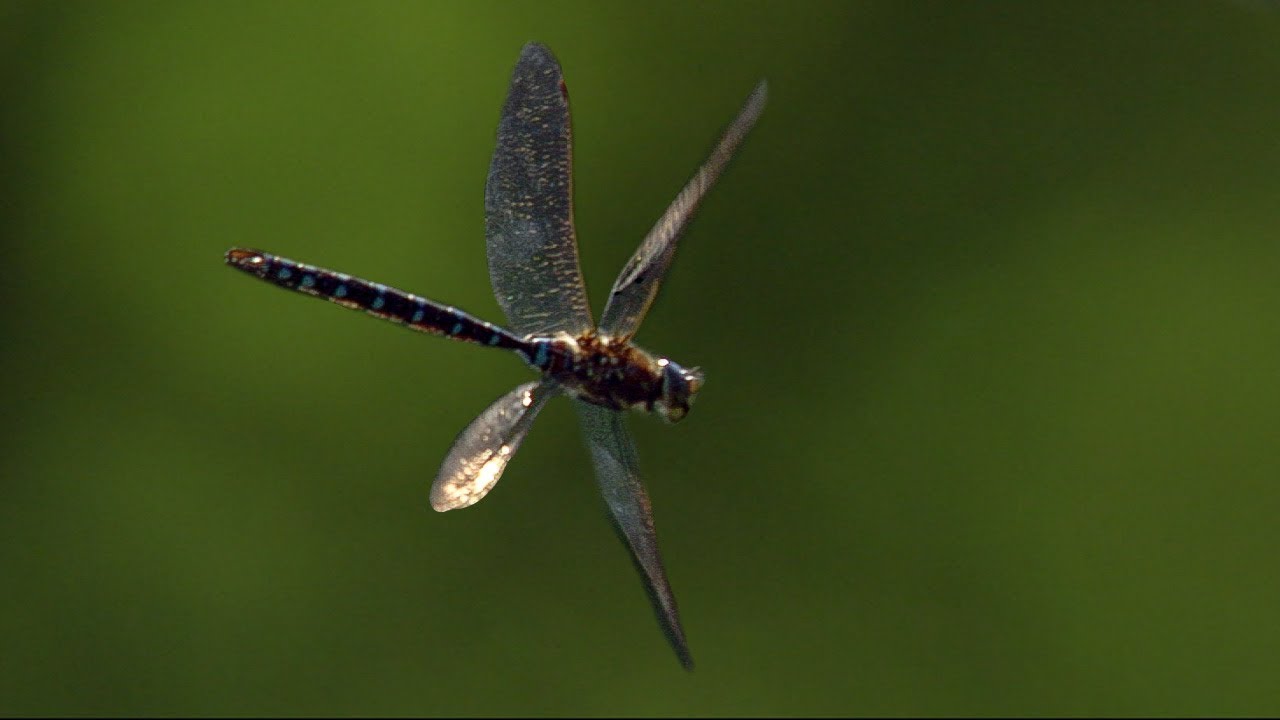In this captivating close-up photograph, we see a dragonfly mid-flight against a blurred, green outdoor background. The dragonfly's four translucent wings, arranged in an X shape, display accents of grey, white, and goldish-brown with hints of orange. The upper left wing appears notably wider and the bottom left wing shorter, likely due to its angled posture as it flies to the right and slightly away from the viewer. 

The dragonfly's head features a mix of blue and brown with light yellowish or brownish eyes. Its body is darkish brown with a hairy texture just below the head, transitioning to a long, slender tail marked by stripes of black and blue. The tail, extending longer than the combined length of the head and torso, showcases seven distinctive light blue spots. This detailed image highlights the delicate and intricate beauty of the dragonfly's features against the green-toned, out-of-focus backdrop.